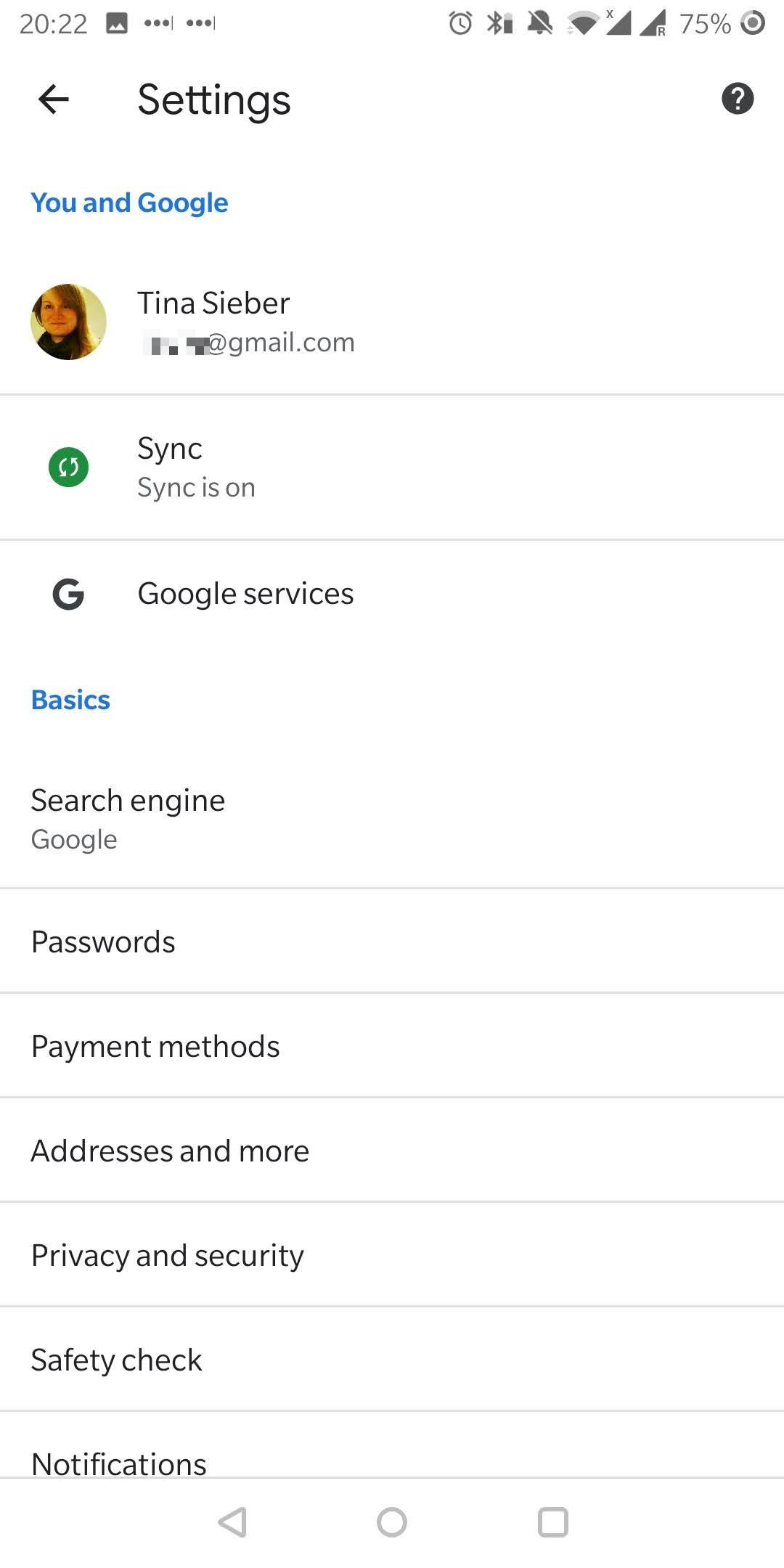This image showcases a screenshot of a mobile screen, specifically within the settings tab, providing a detailed look at various on-screen elements. In the top left corner, the time is displayed as 20:22. Adjacent to the time are three icons: a black square with two small triangular mountains at the bottom, an icon with three dots connected by a line, and a duplicate of this icon.

Moving towards the top right, there's the letter 'A,' followed by several status icons: an alarm clock, a white Bluetooth signal, a bell with a line through it, a signal strength icon (half full), a shaded triangle with an 'X,' another shaded triangle with an 'R' inside, a battery indicator at 75%, and a dot encircled.

Below this status bar, on the left side, is a backward arrow next to the word "Settings." On the right side of this same row is a black circle containing a white question mark.

The subsequent section's heading, "You and Google," is highlighted in bold blue letters. Below this heading is a profile photograph of a Caucasian woman with long, shoulder-length brown hair identified as Tina Sieber, followed by her partially obscured email address ending in @gmail.com. 

A gray horizontal line separates this section from the next, which indicates the synchronization status with "Sync is on" marked next to a green dot encompassing a circular arrow representing sync.

Another gray line divides this portion from the next area, displaying the Google 'G' logo with the label "Google services" beside it. Under the "Basics" heading in bold blue, the options listed include "Search engine (Google)," "Passwords," "Payment methods," "Addresses and more," "Privacy and security," "Safety check," and "Notifications."

At the bottom of the mobile screen are three navigation icons: a backward arrow, a circle, and a square.